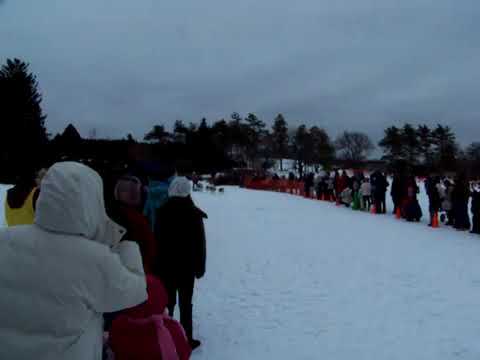A color landscape photograph captures a snowy outdoor scene during the Iditarod sled dog race in Alaska. In the foreground, numerous spectators, clad in heavy jackets, parkas, and hoods, stand in the snow, eagerly watching the race. On the left, a person in a white jacket with a white hood stands beside another in black with a white hat, while another, donning a black jacket with a yellow vest, stands further along. Cones are set on the snow to keep the onlookers at bay. On the right, more people line up along the snowy path, which carves a white, pristine opening for the incoming sled. Just behind the spectators, a team of sled dogs is seen pulling a sled, their figures tiny in the distance and blurry upon closer inspection. The backdrop features a row of mostly dense evergreen trees, except for one barren tree devoid of leaves. Overhead, the sky presents a gray, stormy hue, contributing to the photo's dark and hazy aesthetic. The image authentically captures the anticipation and chill of the race event in a representational and realistic style.